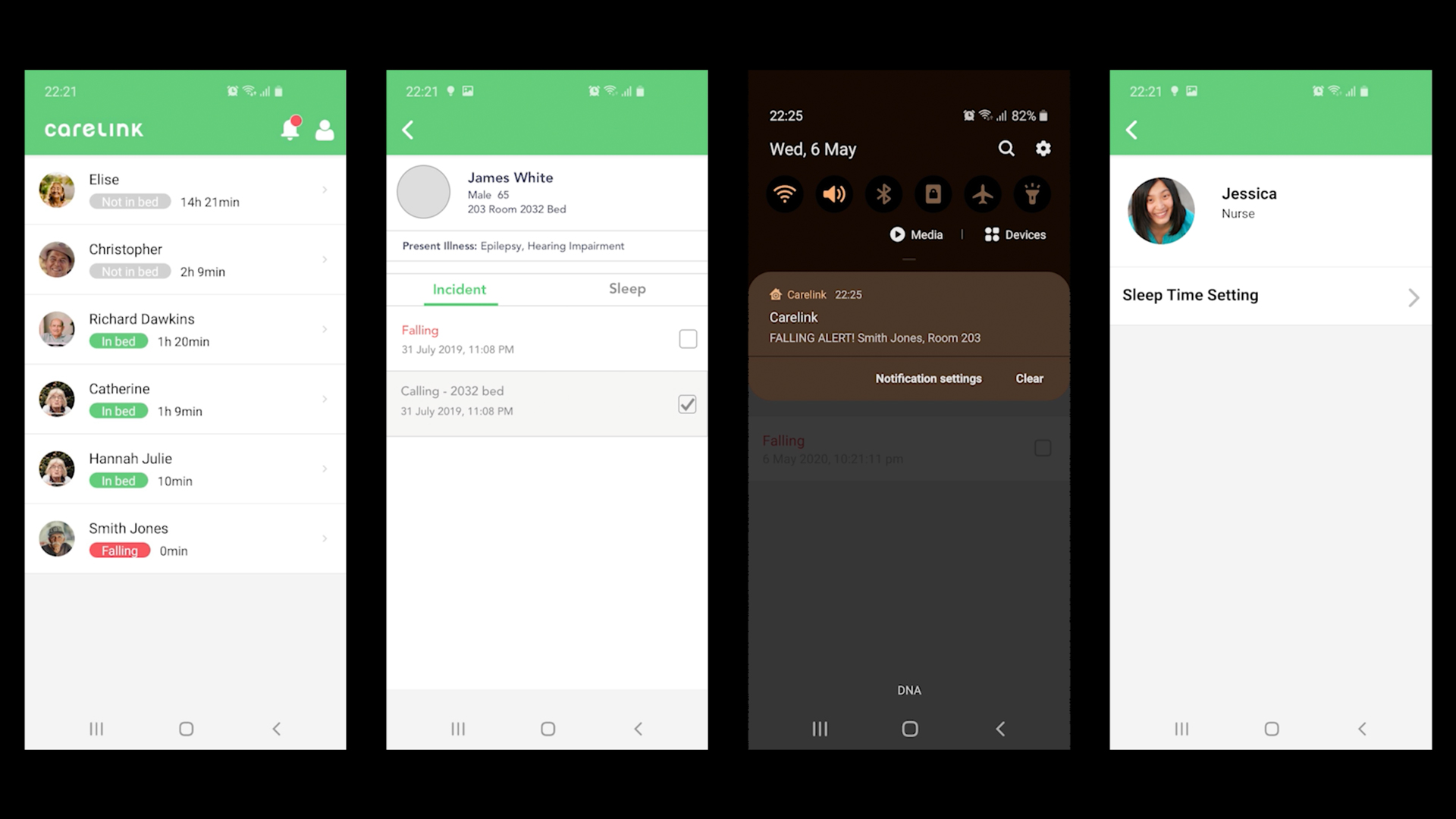In this image, there are four screenshots arranged against a black background.

**Top Left Screenshot:** The top left corner displays the time as 12:21. Directly below, there is a green banner labeled "Care Link." To the right of the banner, notification icons are visible. The upper right corner shows full Wi-Fi signal bars and a fully charged battery indicator.

**Top Right Screenshot:** This section contains details on several individuals in a column format. First is "Elise," accompanied by a small image of a woman. It reads "14 hours 21 minutes, not in bed." Next is "Christopher," noted as "not in bed, two hours nine minutes." Following is "Richard Dawkins," highlighted in green with white text in a box, stating "in bed, one hour 20 minutes." Lastly, "Catherine," depicted as an older woman with gray hair, is listed as "in bed, one hour nine minutes."

**Bottom Left Screenshot:** Below the green banner, this screenshot begins with the profile of "James White," a 65-year-old male, located in room 2032, bed 2032. His present illnesses are listed as epilepsy and hearing impairment.

**Bottom Right Screenshot:** This section contains brief entries labeled "Incident" and "Sleep," though their detailed descriptions are not fully visible in the provided context.

The cohesive layout provides a comprehensive overview of patient statuses and personal details within the given care system.